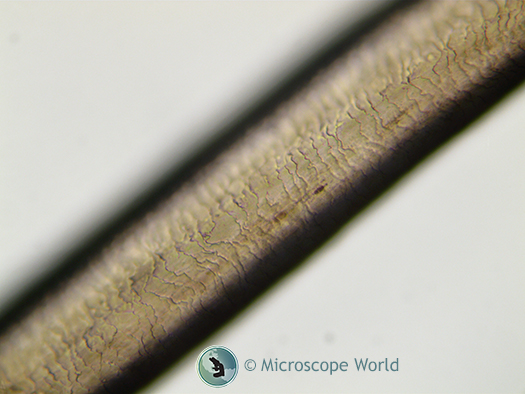This is a detailed microscopic image, approximately nine and a half inches wide by seven inches tall, set against a light grey, almost bluish white or grayish white background. At the center of the image, running diagonally from the upper right-hand corner to the lower left-hand corner, is what appears to be a magnified strand of hair or possibly a microscopic tubular sample of a plant. The central object is light brown with several cracks and irregular wrinkles or creases, reminiscent of dry skin. There are also slight highlights of pale yellow and darker brown slashes on its surface, with notable shadows to the left and right giving it depth. At the bottom of the image, there’s a logo featuring a green circle resembling the Earth, with a silhouette of a microscope inside it. Alongside this logo are the words "Microscope World," signifying the image’s origin.